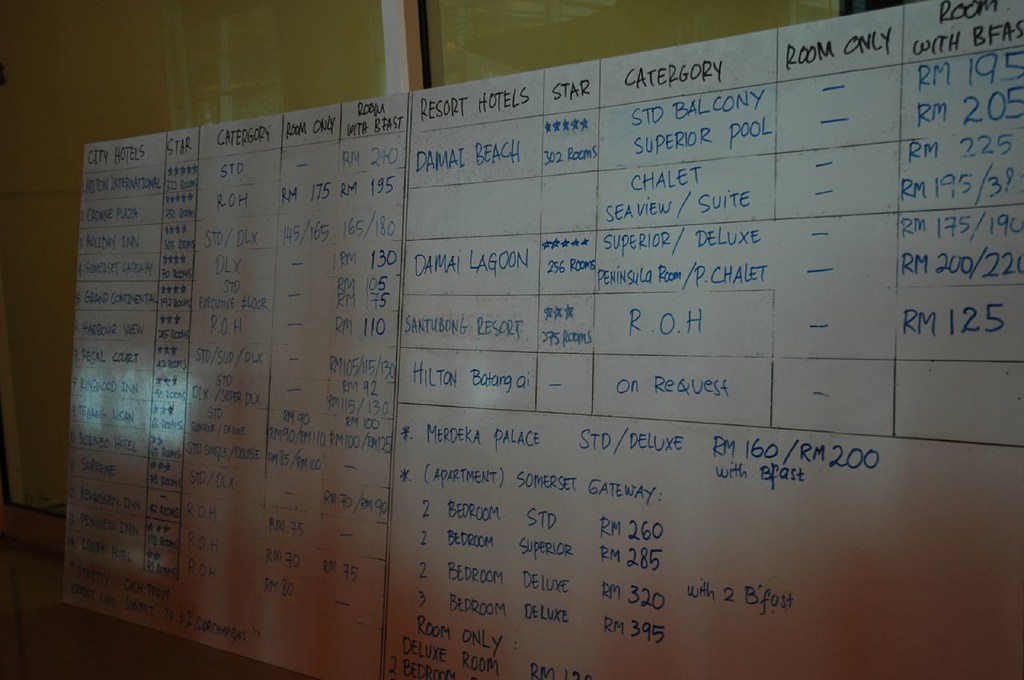This photo captures a large, shiny whiteboard divided into two main sections by black vertical and horizontal lines, creating organized boxes. The whiteboard is set against a greenish wall in a dimly lit room, with reflections from opposite windows faintly visible on its surface. 

On the left section, the whiteboard lists various city hotels categorized by star ratings, number of rooms, room types, and pricing. For example, the Hilton International is noted as a 5-star hotel with 322 rooms offering standard categories; room only rates are blank, while rooms with breakfast cost RM240. Several other hotels like Ocean Plaza, Holiday Inn, Somerset Gateway, Grand Continental, and others are systematically detailed with similar information, including specific prices for different categories such as standard, deluxe, executive floors, etc.

The right section is dedicated to resort hotels. Each resort is rated by stars and details its room types and associated costs. For instance, Damai Beach Resort is a 5-star resort with 302 rooms in various categories like Standard Balcony, Superior Pool, and Sea View, among others. Prices for rooms with breakfast range from RM195 to RM390, while room-only rates are blank. Other resorts listed include Damai Lagoon, Shantubong Resort, and Hilton Resort AI, with specific details about their room types and rates.

There are also supplementary details and footnotes regarding additional charges and room categories such as the Madhya Palace and Apartment Somerset Gateway, with various room types and breakfast inclusions.

Overall, the whiteboard provides a comprehensive comparison of hotel and resort options, meticulously detailing their star ratings, room categories, and pricing structures.